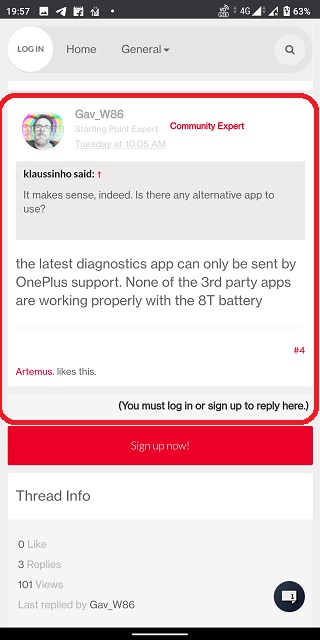A screenshot from a mobile device displaying a forum thread, indicated by visible elements such as the time and battery life at the top. The interface includes a circular home button, a dropdown menu, and a magnifying glass icon for search functionality. 

Highlighted in a prominent red-bordered box is a user named "gav_w86," identified as a community expert. Below his name, user "colanzo" comments, "Makes sense indeed. Is there any alternative to app to use?" This text is encased in a grey box. The response details: "The latest diagnostic tab can only be set by OnePlus support. None of the third-party apps are working properly for the battery."

Artemis has endorsed this post, noted by "Artemis likes this" in red, followed by "#4." An invitation to "log in or sign up to reply here" is shown in parentheses, prominently underlined with "sign up now" in red text. 

The thread information is displayed next, showing bold counts for "0 likes," "3 replies," and "101 views." The thread's latest interaction was by "gav_w86." To the right, a comment icon invites additional remarks.